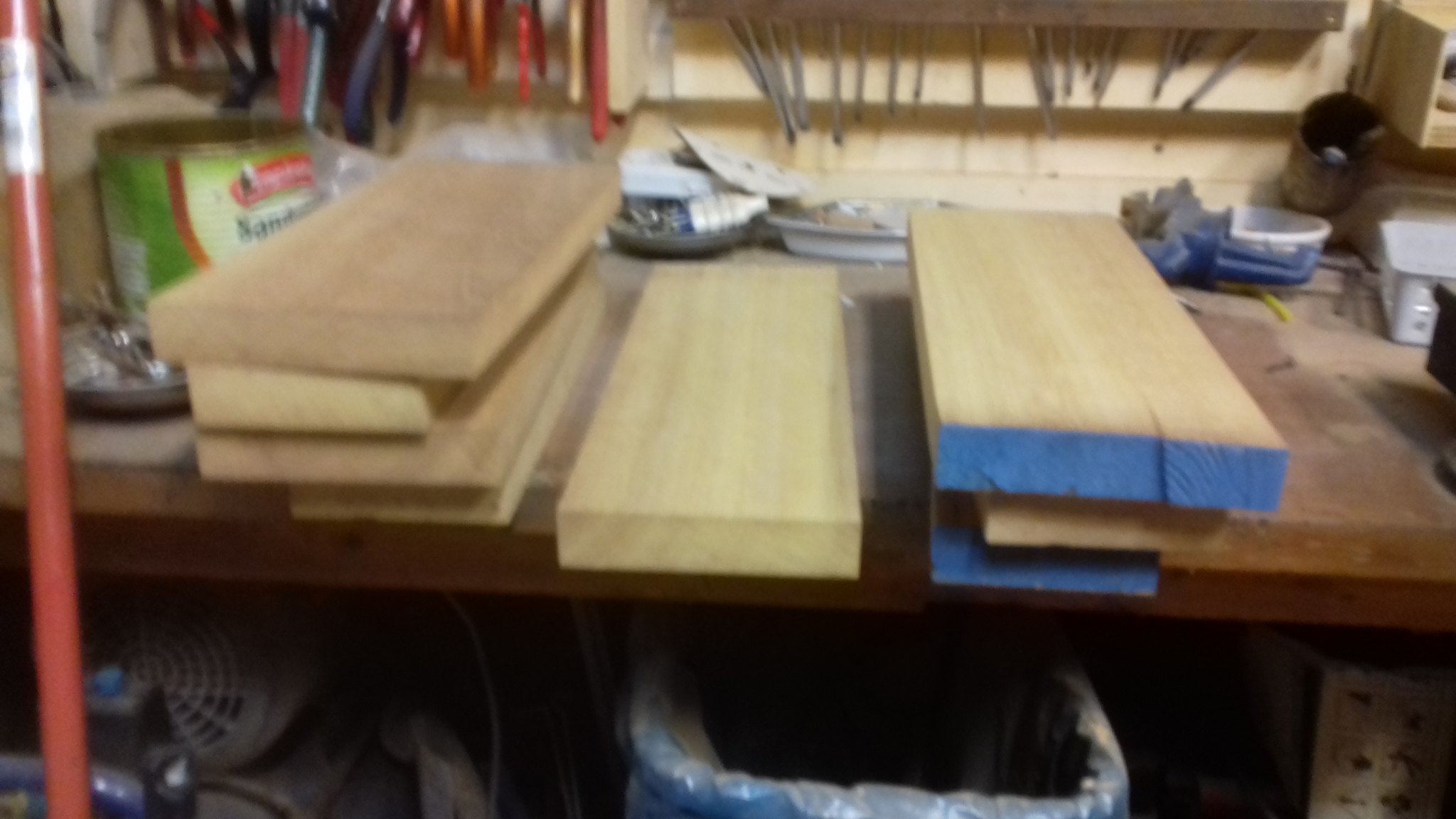The image captures a well-used wooden workbench in a cluttered garage or workshop. The workbench itself bears the marks of labor, with various nicks and scars on its surface, covered in layers of sawdust. On the bench lies an assortment of cut lumber, primarily 2x4s of varying lengths. On the left side, a stack of four boards is visible, with a solitary board in the middle and a stack of three on the right. Notably, the boards on the right have their ends painted blue. Below the bench, a blue trash can is situated directly underneath, accompanied by a collection of tools including fans and a metal can without a lid. 

In the background, the wall is lined with an array of hanging tools such as pliers and screwdrivers, with their handles prominently visible. These tools range in size and type, forming a continuous line across the wall. On the workbench surface are various dishes, bits of paper, small cups, and indeterminate items due to the low resolution and graininess of the picture. To the left, there is an open metal can and what seems to be a broom handle. Adding a unique touch, a cat photobombs the bottom left corner of the frame, its eyes glowing due to the camera flash. Despite the blurriness and grainy quality of the photo, the scene vividly conveys the busy, practical atmosphere of a working garage or workshop.